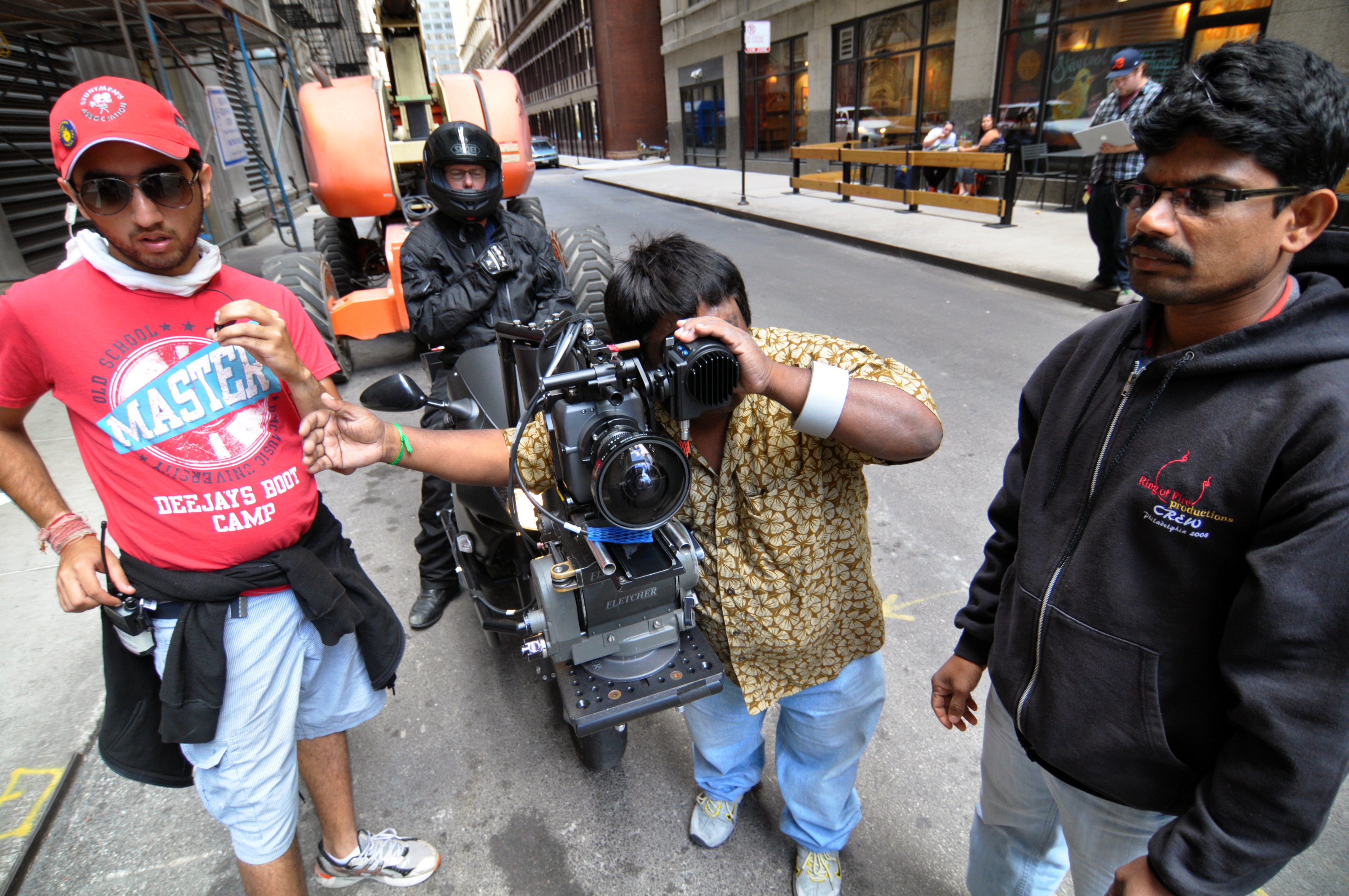In this vibrant city street scene, four individuals are conspicuously occupied in what appears to be a filming project. Situated at the center of the drama, a cameraman, potentially the director, is engrossed in capturing the perfect shot with a large camera, likely affixed to a sophisticated crane system. His frame is small, possibly suggesting he is of Asian descent, and he is adorned with a white bracelet on the wrist that manipulates the viewfinder. Standing to his left, engrossed in his role with sunglasses on, is a man in a red t-shirt and cap, with a black sweater tied around his waist, and blue shorts; he's fiddling with a walkie-talkie strapped to his hip.

On the right side, another man, distinguishable by his black zip-up sweater, glasses, moustache, and blue jeans, appears contemplative, gazing downward. Behind this engaging tableau stands a person on a moped, dressed in a motorbike helmet and jacket, likely responsible for maneuvering the mobile camera rig.

The backdrop features high-rise city buildings, with outdoor cafes where diners are engrossed in meals, and scaffolding on a nearby building contributes to the urban charm. The whole setup exudes a sense of dynamic collaboration and captures a slice of life in the bustling heart of the city.